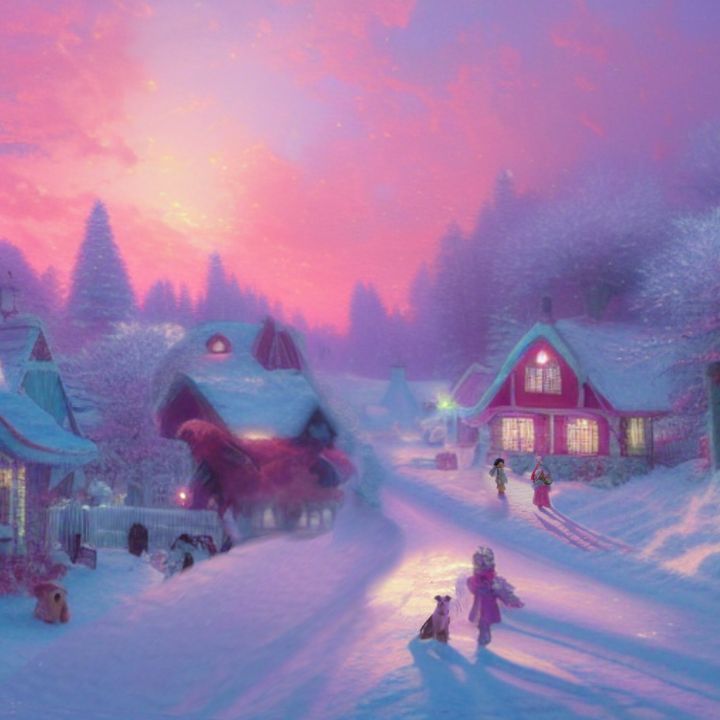This detailed descriptive caption combines elements and details from all three captions provided:

The scene depicts a painting with an impressionistic style featuring a small, wintry village reminiscent of a Christmas card. Broad brush strokes illustrate snow-covered houses and trees, casting a serene atmosphere. We observe the village from an elevated perspective, almost as if looking down from a rooftop, capturing the charming essence of this quaint snow-filled town. Three houses, identifiable by their glowing windows and red peaked roofs, are decorated with Christmas lights. The snow-covered streets form a Y-intersection, where a young girl stands alongside her dog, framed perfectly in the foreground. Off to the right, two children, dressed warmly in scarves with one wearing a green outfit paired with a pink skirt, engage in winter activities. The sky, painted in shades of orange and pink, hints at a setting sun behind the clouds, casting a warm glow over the idyllic scene. Christmas trees dot the background, completing this picturesque holiday setting.